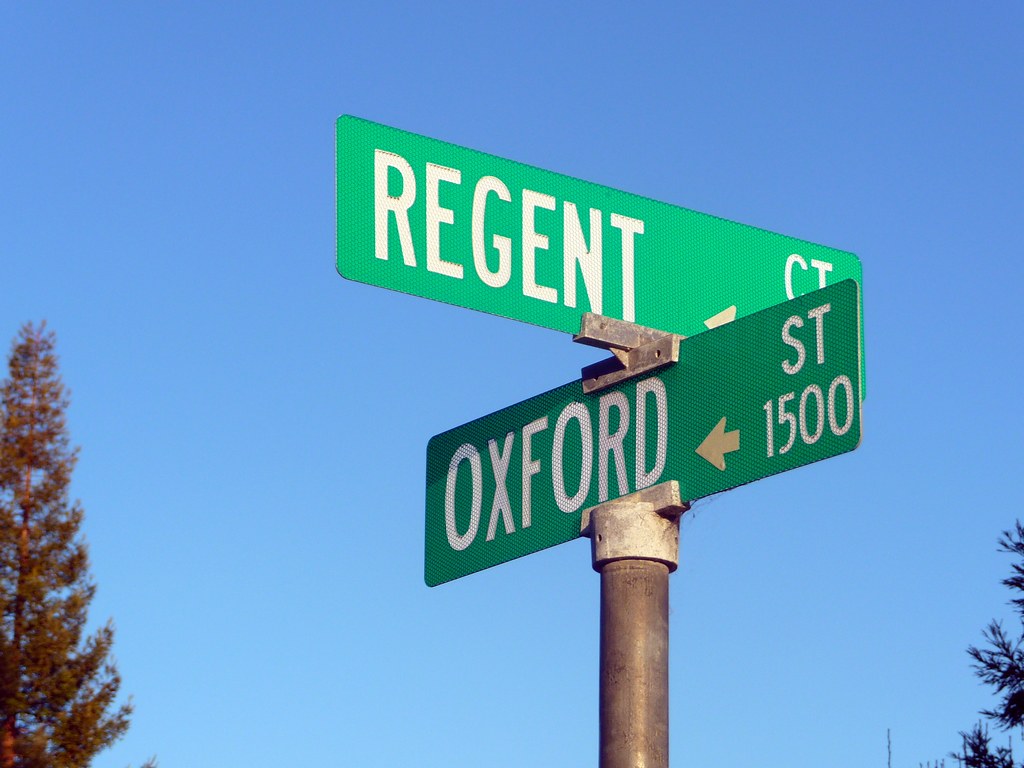The close-up photo showcases a green street sign pair in a neighborhood, mounted on a weathered, white circular post. The sign in the foreground reads "Regent Court" in crisp white lettering, while the intersecting sign beneath it says "Oxford Street 1500," accompanied by a directional arrow pointing left. Despite the aged post, the signs remain well-maintained and intact. The background reveals a clear blue sky flanked by two types of pine trees: a tall, spiky pine on the left bathed in sunlight and a pine with looser branches situated in the bottom-right corner.